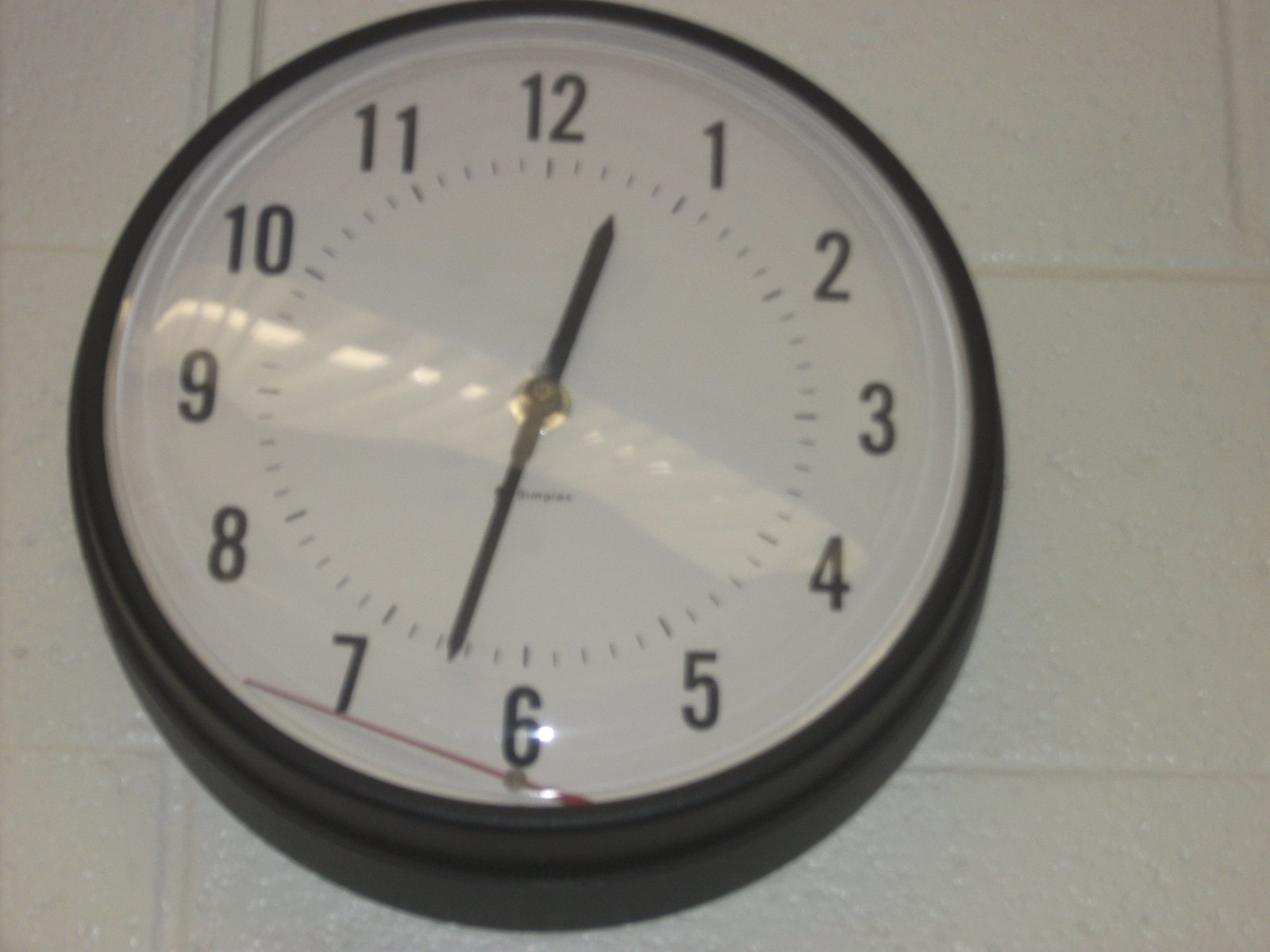This is a close-up photograph taken indoors of a clock mounted on a painted white cinder block wall. The bricks are large and rectangular, uniformly coated with glossy white paint. The clock has a black circular rim encasing a white face with simple black Arabic numerals from 1 to 12. Minute markers are small black dashes around the edge of the clock face. The hour and minute hands are black, rectangular, and ending in points, with the hour hand being shorter and thicker. The time displayed is approximately 12:33, with the hour hand halfway between 12 and 1 and the minute hand between 6 and 7. A brass-colored fastener is at the center of the clock. Notably, the red second hand has broken off from the clock's mechanism and rests inside the glass cover at the bottom, angled between the 6 and 7 positions, giving the clock a slightly broken appearance.